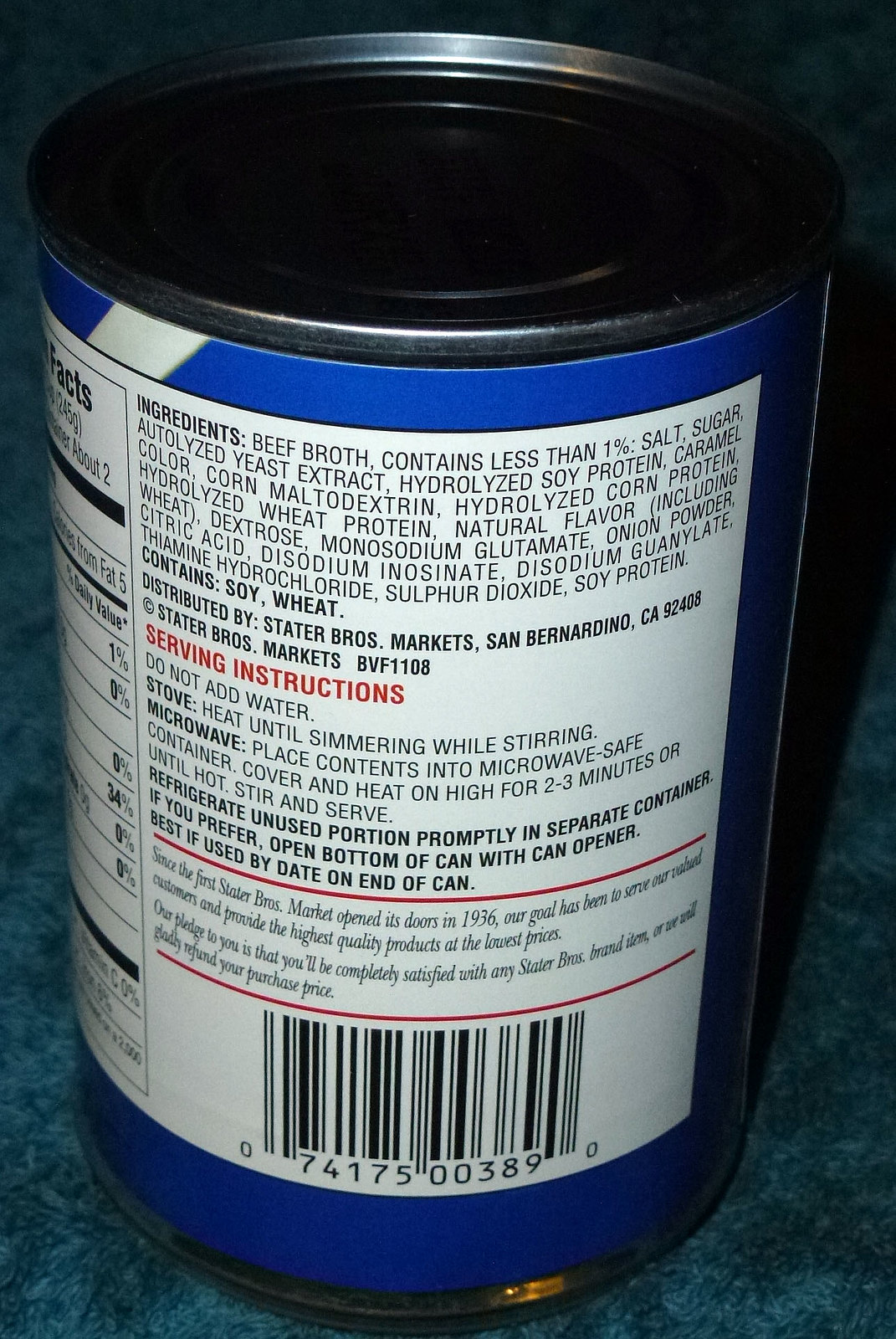The image depicts a vertically aligned photograph of a round, silver, unopened can of food sitting on a blue and black marbled carpet. The primary focus is on the can, which features a detailed label. The label, bordered in blue at the top and bottom, is predominantly white with black text. The label displays ingredient information including beef broth, autolyzed yeast extract, hydrolyzed soy protein, caramel color, cornmeal, and maltodextrin. An instruction section in red letters says "Do not add water, stove, heat until simmering while stirring." The label also includes nutritional values on the left side and a barcode at the bottom.